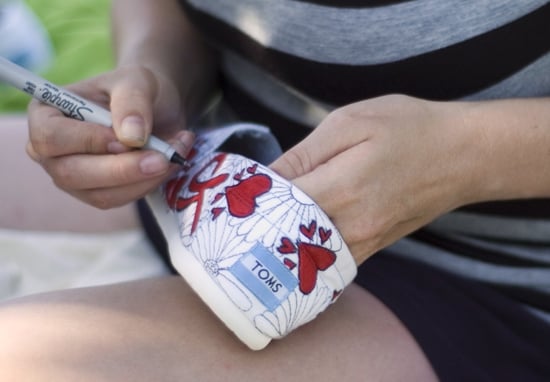In this close-up photograph, a light-skinned individual is seated and intensely focused on decorating a white TOMS slip-on shoe, which rests atop their upper thigh. The person is adorned in a gray and black striped shirt with shorts, and their left hand secures the shoe while the right hand expertly wields a fine-point Sharpie marker, visibly labeled "Sharpie." The shoe brims with intricate black outlines of daisies and hearts, some of which have already been colored red. The individual is in the midst of carefully outlining a red shape, adding to the vibrant, detailed design. The scene captures a moment of artistic creativity, where the simple canvas of a shoe is transformed into a lively tapestry of flowers and hearts through precise, passionate strokes.